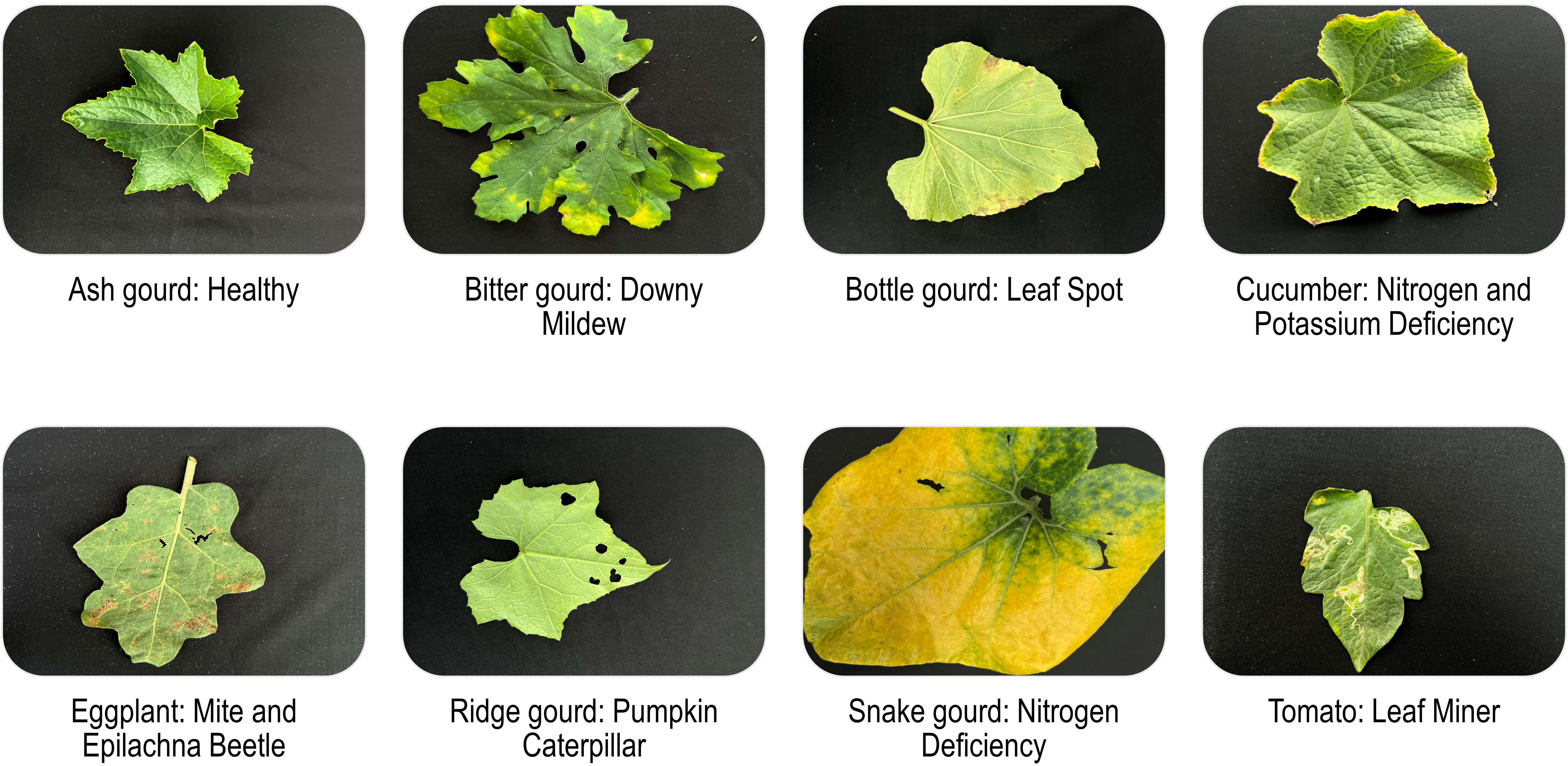The image is a detailed collage of eight distinct leaves, organized in two rows of four. Each leaf has accompanying text in a sans serif font that identifies the leaf type and its condition or associated pest problem. The top row starts with an entirely green leaf labeled "ash gourd, healthy." Next, a slightly larger leaf labeled "bitter gourd, downy mildew" is edged in lighter green. To its right, a lighter leaf identified as "bottle gourd, leaf spot" follows. The next leaf, labeled "cucumber, nitrogen and potassium deficiency," has a textured appearance. In the bottom row, we begin with a leaf that shows brown spots and tears, marked "eggplant, mite, and epilachna beetle." Adjacent to it is a hole-ridden but otherwise healthy leaf labeled "ridge gourd, pumpkin caterpillar." Following that is a predominantly yellow leaf with some green, labeled "snake gourd, nitrogen deficiency." The final leaf on the bottom right is mostly green with noticeable yellow spots, identified as "tomato, leaf minor." This comprehensive display highlights various plant conditions and pest issues, predominantly focusing on gourd family leaves.